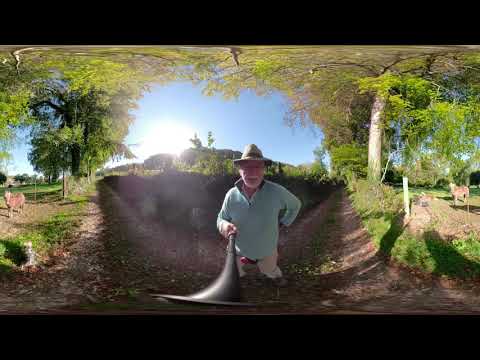This detailed selfie captures an older gentleman, likely in his late 60s to early 70s, standing at the precise fork of a dirt road that stretches out in a pastoral, tree-lined area. He sports a prominent white beard and a wide-brimmed hat that leans towards a cowboy or Indiana Jones style, adding a rustic touch to his appearance. Clad in what appears to be a gray or green zip-up sweater and potentially tan pants, he exudes a sense of ease and familiarity with his surroundings, suggesting a deeper connection or prolonged experience in this natural setting. The image, taken with a selfie stick and somewhat distorted by a fisheye lens, shows the man amidst clear, sunny skies with no clouds, lending a bright and open ambiance. Surrounding him, sparse patches of grass, scattered trees, and possibly crops or animals point towards a farm-like environment. The gentleman appears comfortable and assured, embodying a serene blend of age, wisdom, and contentment as he stands at the crossroad, possibly hinting at both a literal and metaphorical journey.